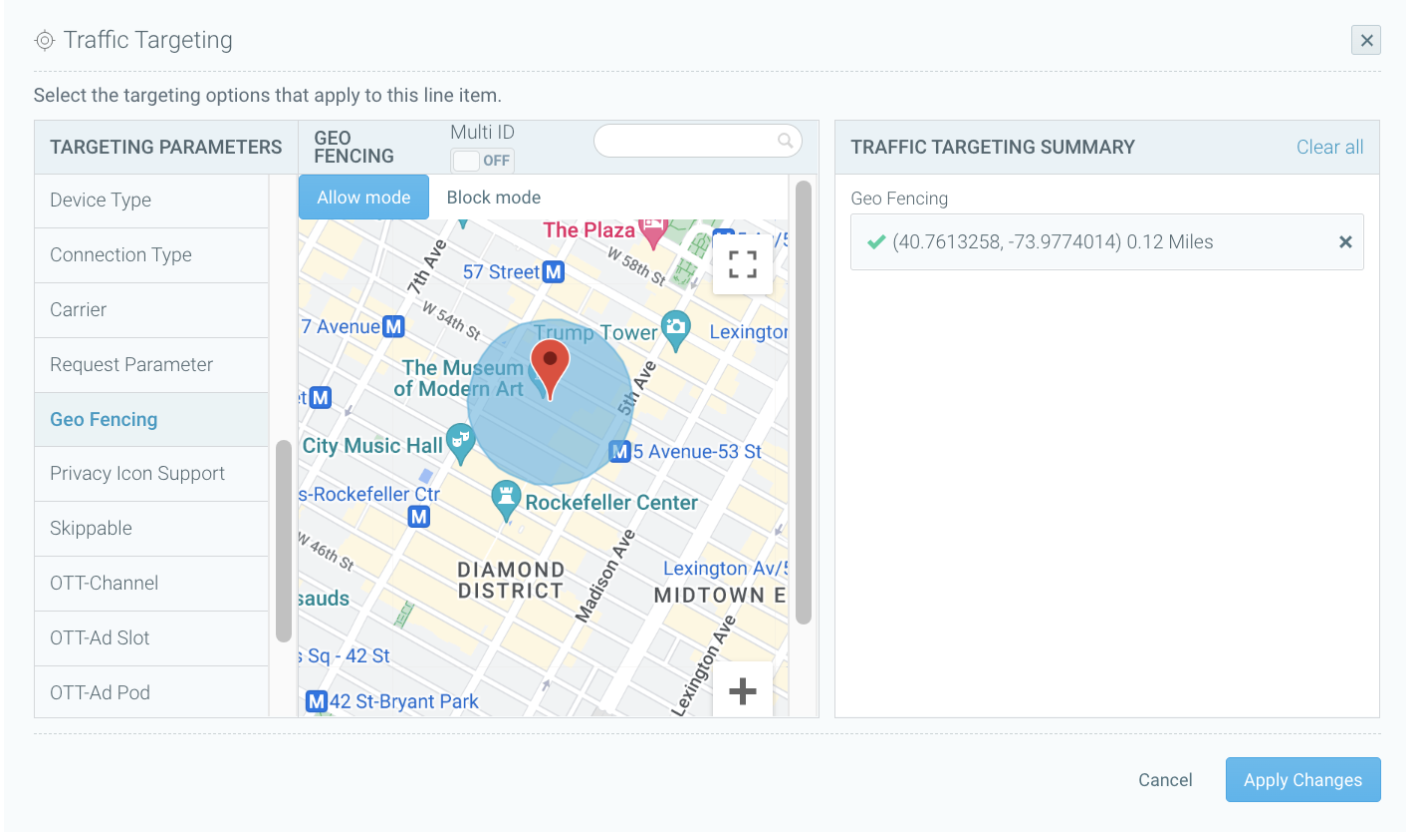This image is taken from a web page related to traffic targeting. The background of the page is a very pale blue. In the top left corner, "Traffic Targeting" is written in gray text. Beneath this heading, there is a smaller gray text instructing, "Select the targeting options that apply to this line item."

On the left side of the page, a vertical list of targeting parameters is displayed. The parameters include Device Type, Connection Type, Carrier, Request Parameter, Geo Fencing, Privacy Icon Support, Skippable, OTT Channel, OTT Ad Slot, and OTT Ad Pod. To the right of this list is a gray scroll bar for navigating through these options.

Geo Fencing has been selected from the list, and accordingly, an interactive map appears to the right side of the page. The map depicts what appears to be a downtown district, likely in New York City. Featured on the map is a wide blue circle with a red location icon at its center, illustrating the targeted area. Landmarks identified on the map include Rockefeller Center, Midtown, the Diamond District, and Radio City Music Hall.